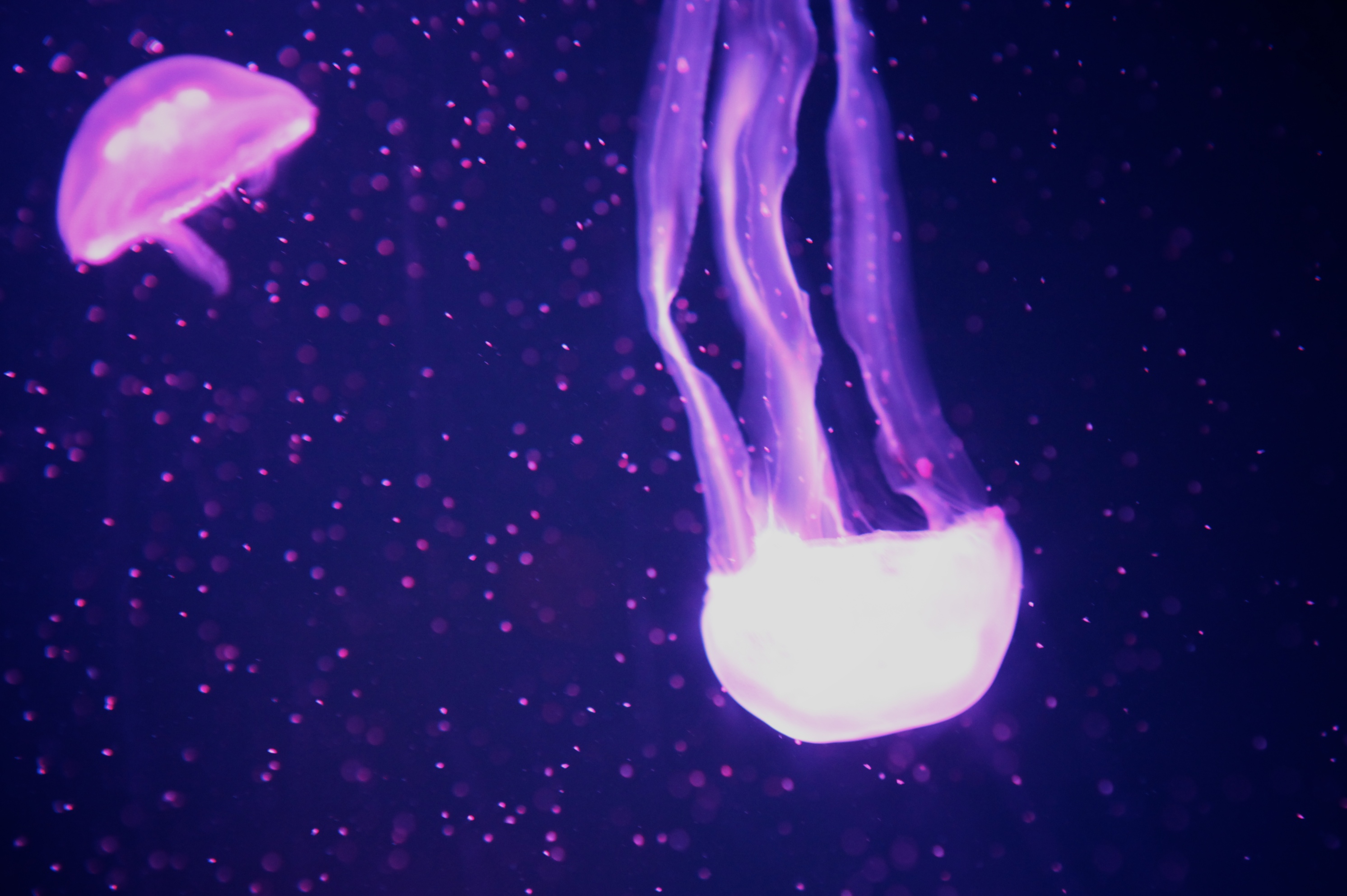This surreal, possibly computer-generated image features two luminescent jellyfish against a predominantly black background sprinkled with delicate, glowing specks of purple. The larger jellyfish occupies the foreground, its bright white mantle tapering downwards with three delicate, trailing tendrils that stretch upwards. These tendrils are semi-translucent, a blend of dark and light purple, and give off an appearance reminiscent of lightning. The dome-like mantle also has subtle hints of purple around its edges, emphasizing its ethereal glow. In the top left corner, a smaller jellyfish floats with its mantle pointed upwards. It has a pinkish hue and its tentacles are much shorter and less distinct than those of the larger jellyfish. Its mantle also exhibits a pink to purple gradient, blending seamlessly into the dreamy atmosphere. The background is an enchanting mix of deep blacks interspersed with lavender and violet specks, concentrating more densely on the left side of the image. These glowing elements enhance the overall otherworldliness of the scene.